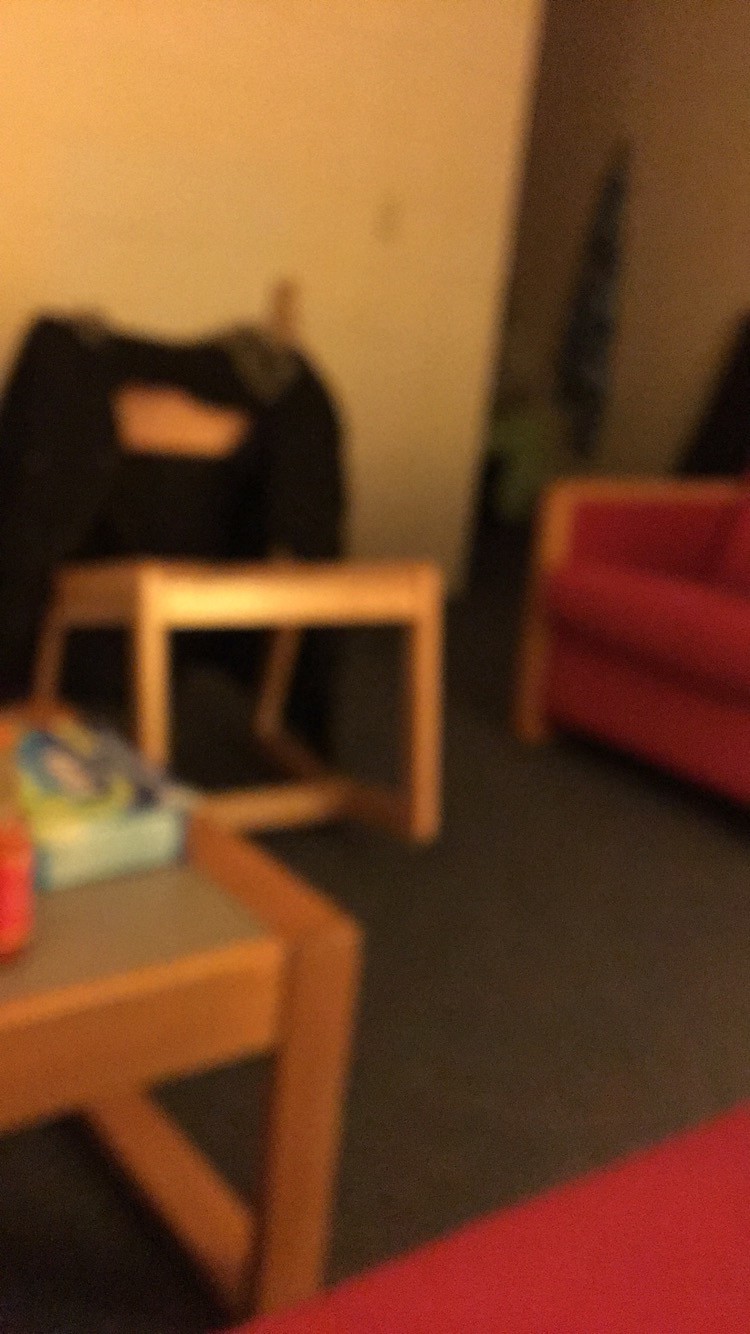This blurry photograph captures an interior living space, potentially a sitting area, with a light yellow wall in the background. On the right side of the image, there appears to be an opening leading to a hallway. Just outside this hallway is a red chair with a visible armrest. Adjacent to the red chair is a wooden rocking chair with a black sweater or jacket draped over its back. Closer to the foreground, there's a wooden side table, which could possibly be an oak surface, with a blue box and what looks like fabric softener sheets or Kleenex on top. The floor is covered with a dark gray, short-haired rug. In the bottom right corner, there is a hint of red material, likely another piece of furniture, possibly a matching couch or sofa to the red chair near the hallway. The overall image is indistinct due to the blur, making finer details difficult to discern.